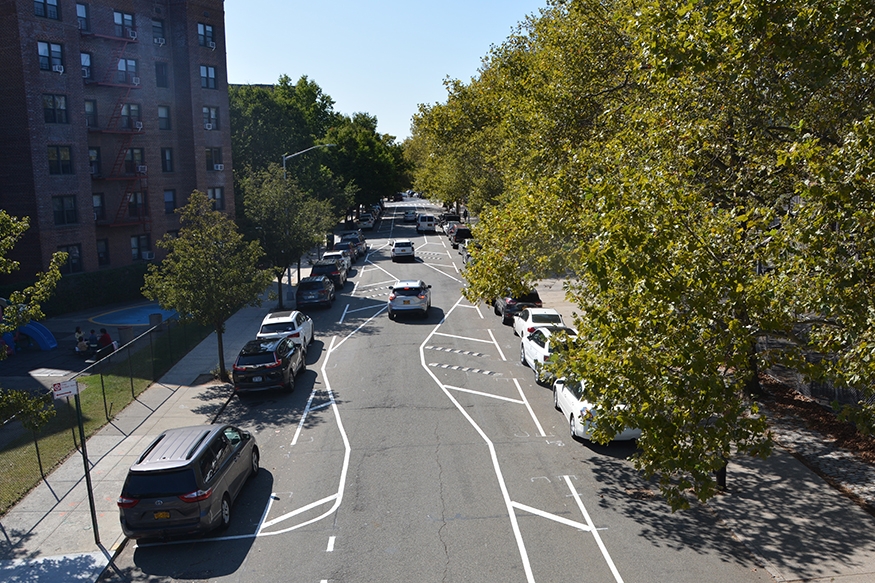This aerial photograph, likely set in a European city, shows a residential street with a distinct zigzag pattern painted onto the road, likely to calm traffic in this neighborhood. The image captures the street from a vantage point several dozen feet above, providing a central view of the road flanked by rows of parked cars. Cars are stationed on both sides of the street, oriented in opposing directions. There are also a few vehicles maneuvering through the zigzag lines. The road features a crosswalk, and the sidewalks on either side host a beautiful collection of trees, particularly dense on the right. On the left, behind a fence, stands a multi-story brick apartment building so tall that its upper stories extend beyond the frame of the photograph. The day is clear with a blue sky free of clouds, adding to the picturesque quality of this residential scene.